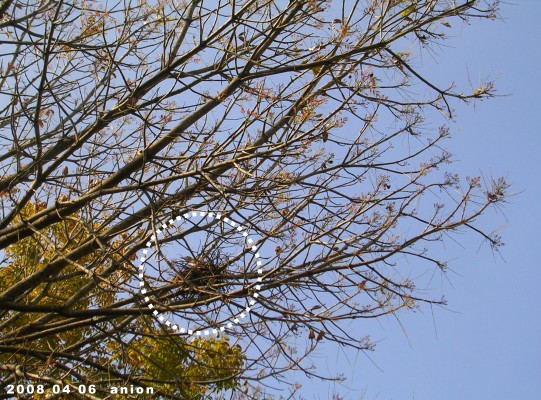The photograph captures a mostly bare tree against a clear, blue sky, with its light brown branches stretching from the lower left-hand corner towards the upper right-hand corner. Small green shoots are visible at the ends of the branches, while numerous small birds are scattered throughout. A dotted, hash-marked circle in the lower left portion of the image highlights a compact bird's nest made of small sticks, nestled close to the bottom of the tree, with a bird peeking out. The background shows another tree adorned with orange and yellow leaves. In the lower left-hand corner, white text is overlaid, reading "2008-04-06 Anon, A-N-I-O-N."